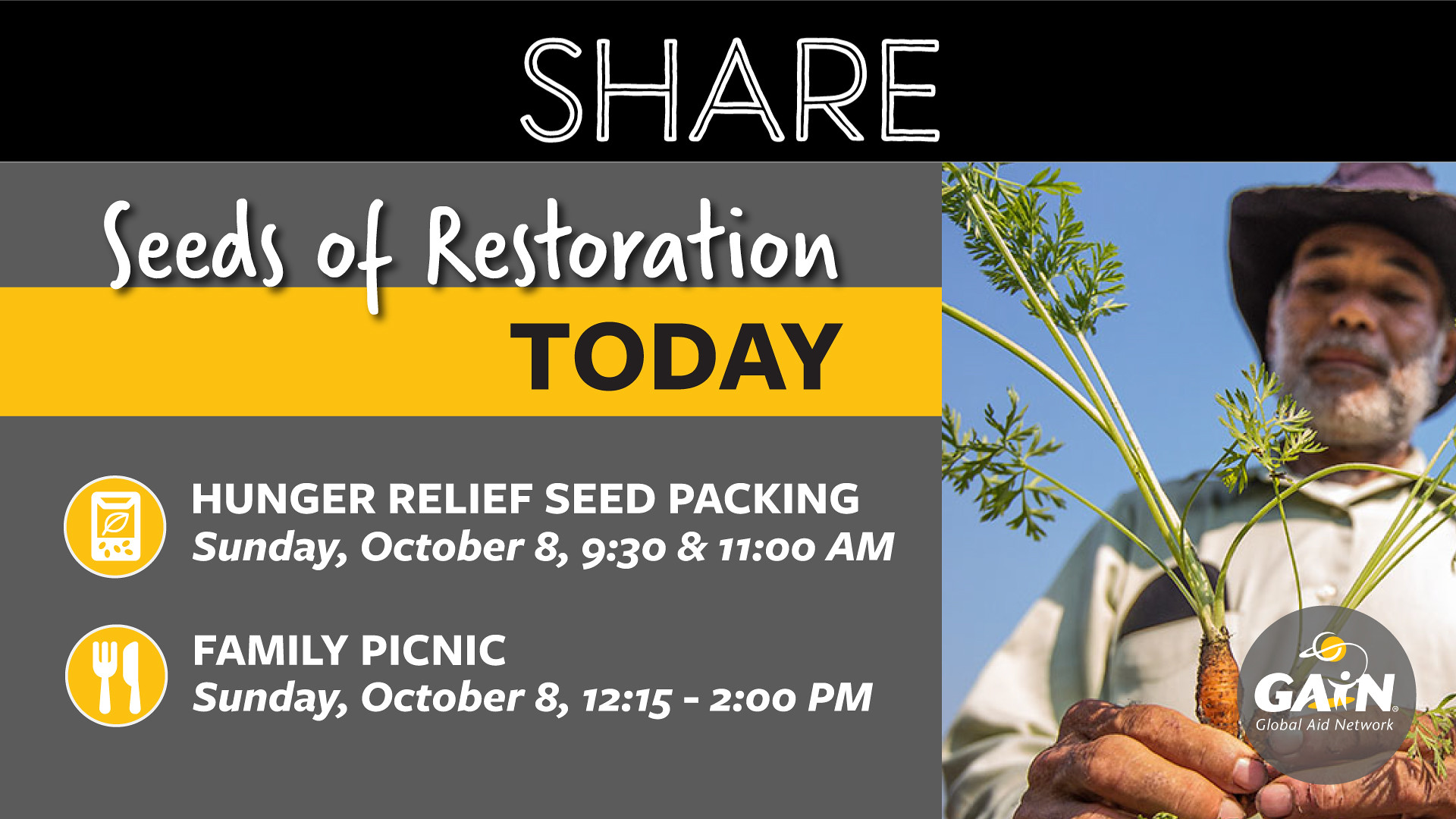This image serves as an advertisement, possibly for a PowerPoint slide or a sign, featuring a detailed event announcement. Dominating the top, "SHARE" is prominently displayed in white capital letters on a black band. Below that, aligned to the left, the text reads "Seeds of Restoration" followed by "Today" on a yellow band. Further details include "Hunger Relief Seed Packing," scheduled for Sunday, October 8, at 9:30 and 11:00 a.m., and a "Family Picnic" on the same day from 12:15 to 2:00 p.m. 

On the right side of the advertising text, there's a poignant image of a black man with a gray beard. He is wearing a tattered black, brimmed hat and a tan button-down shirt with long sleeves. The man is slightly blurry, drawing clear focus to the freshly pulled carrots he holds, which still have their green tops and dirt on them. This imagery is complemented by a logo in the bottom right corner that features a planet and the words "GAIN Global Aid Network."